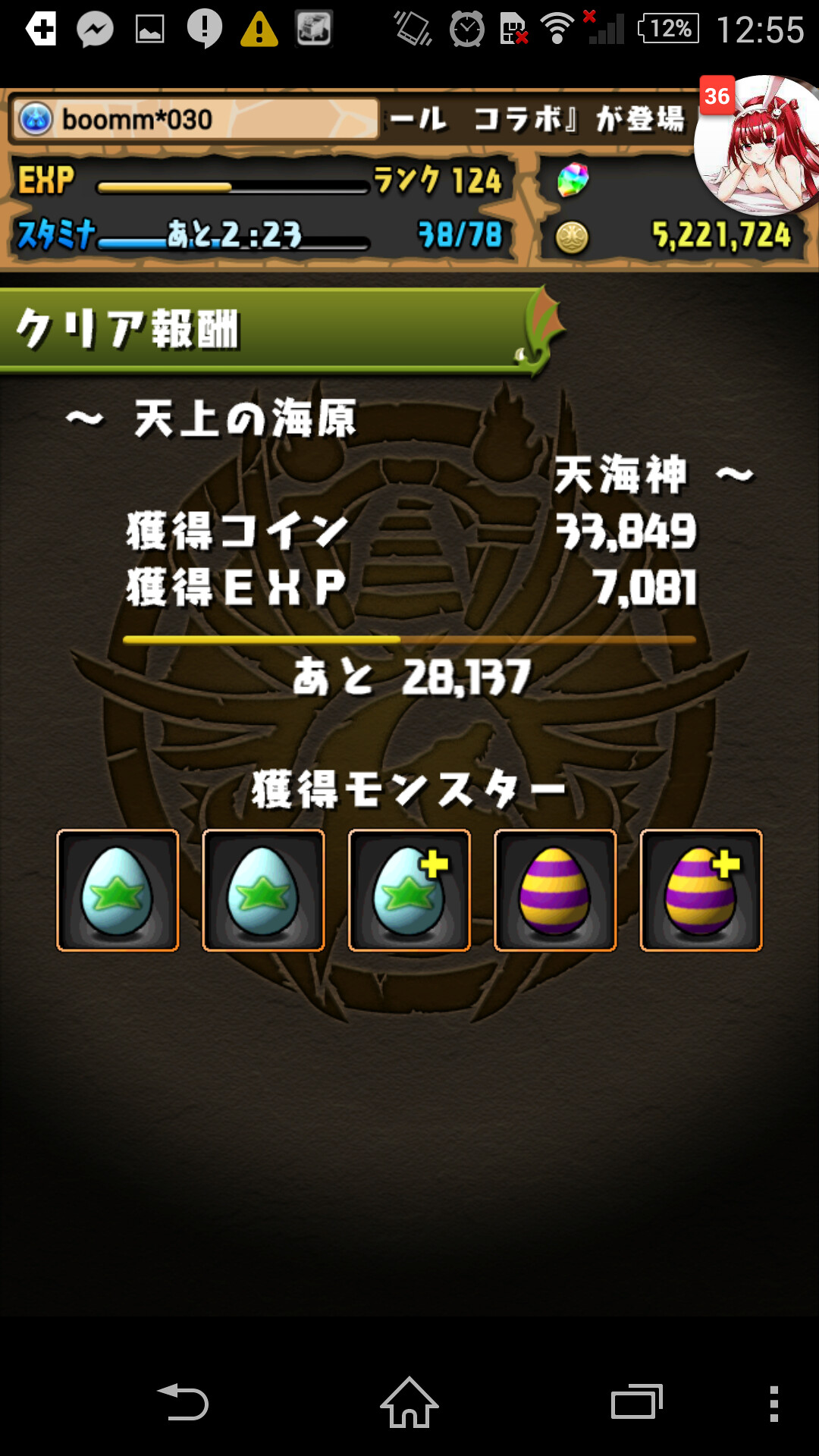This image is a screenshot of a mobile RPG game with various in-game and phone notifications visible. At the top of the screen, there's a yellow experience (EXP) bar accompanied by the username "BOOM*030" beside an avatar of a red-headed anime girl. The avatar displays 36 notifications, likely from multiple sources. The game interface features 5,221,724 gold and 38 out of 78 mana. Most of the game's text is in Japanese. Five egg icons are present at the bottom: three are teal with green stars, and two are yellow with purple stripes, with two eggs marked by a plus star. The background seems to depict a dragon. The phone's status bar shows it has 12% battery left, several power notifications, and a missing SIM card notification. The time displayed is 12:55 PM.